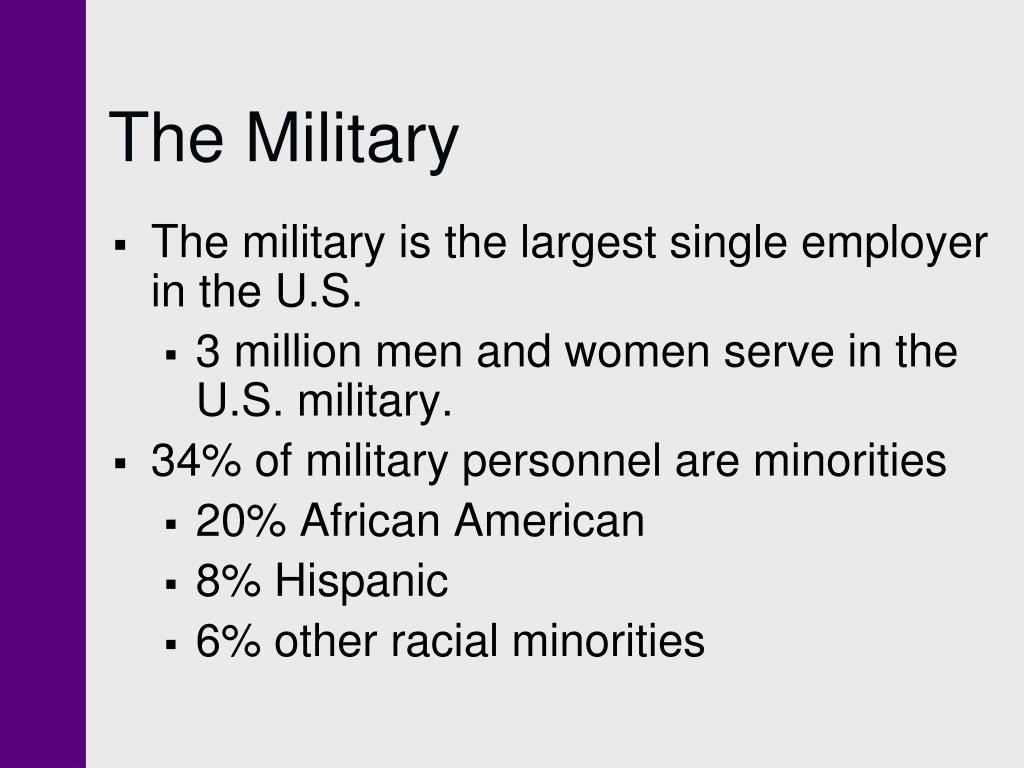The image depicts a straightforward PowerPoint slide designed to present military statistics. The gray background features black text in a printed font, heavily using bullet points to convey the information. At the top of the slide, the title "THE MILITARY" is prominently displayed in capital letters, albeit with a misspelling ("M-I-L-I-T-A-R-E-Y"). The text states that the military is the largest single employer in the U.S., with 3 million men and women serving. It further details that 34% of military personnel are minorities, broken down as 20% African American, 8% Hispanic, and 6% from other racial minorities. A vertical purple stripe on the left side of the slide adds a splash of color to the otherwise minimalistic design.